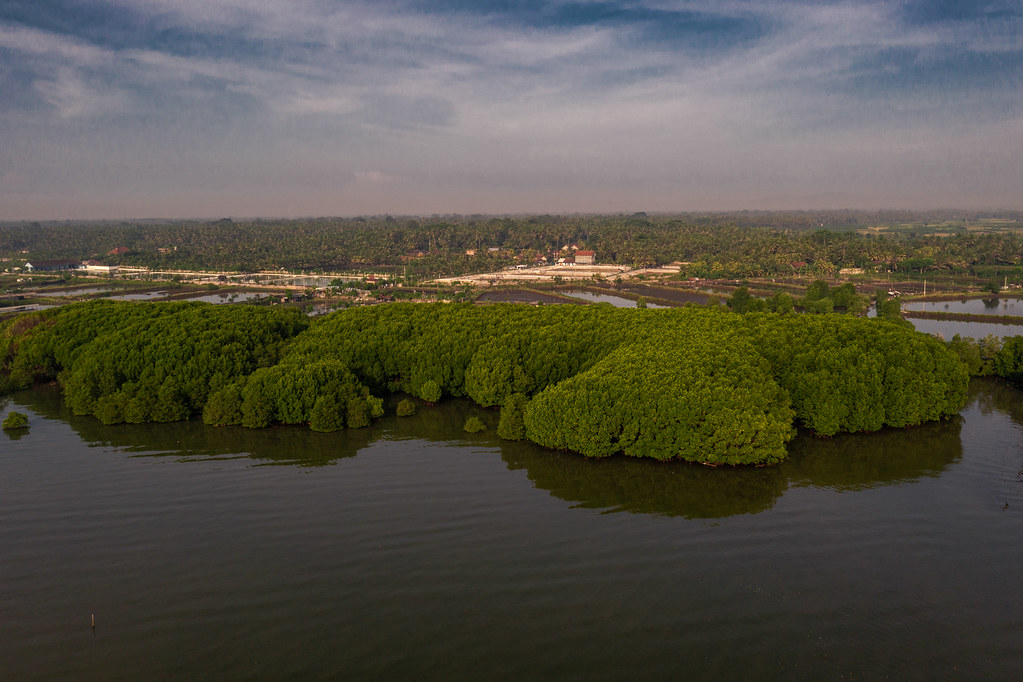This detailed aerial photograph captures a serene, developed landscape, blending natural and man-made elements seamlessly. At the bottom third of the image lies a calm, dark-colored lake or body of water, with barely a ripple disturbing its surface. Emerging from the water is a small, island-like landmass densely packed with tall, green trees, creating the illusion of a steep wall of foliage. This island features several small inlets and appears very lush, resembling a mossy mound rising gently from the water.

Above the island, the terrain transitions into a series of rectangular, silvery water cells separated by small causeways, suggesting rice cultivation or low-lying, flood-prone fields. On the far side of these segmented plots, a developed facility with white buildings and red roofs becomes visible, hinting at human habitation and infrastructure.

Further into the background, a verdant, jungly forest extends along the horizon, with tan-colored fields and more forested areas visible to the right. A few bridges and roads are discernible amidst the greenery and buildings, connecting various parts of the landscape. The horizon itself reveals a subtle pinkish or brownish tinge, gradually fading into a sky filled with wispy white clouds against a backdrop of deep blue.

This image exudes a tranquil yet vibrant scene, capturing the interplay between nature and human development, framed under a partly cloudy, serene sky.